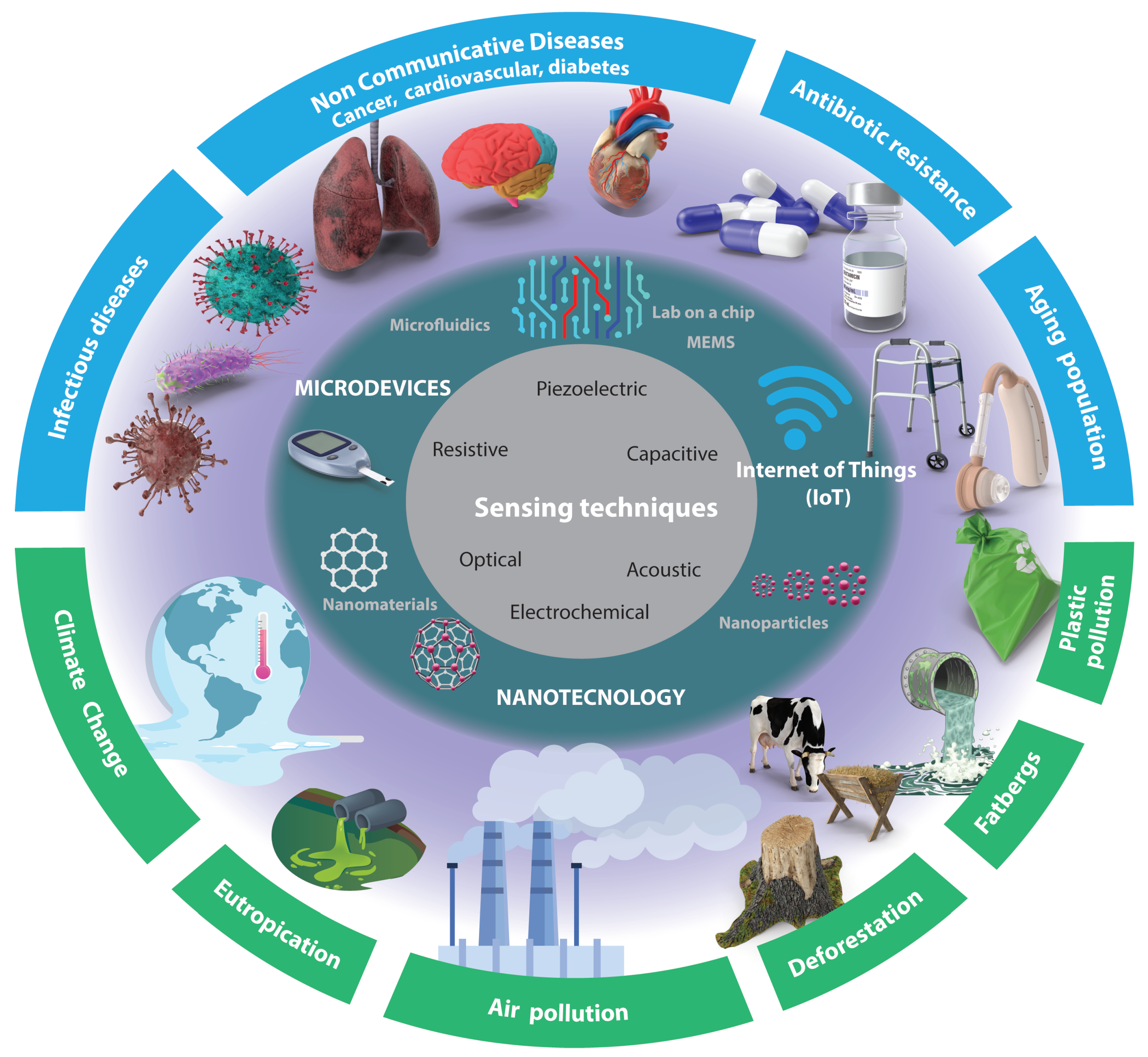The image is a large, detailed circular diagram segmented into various curved rectangular sections and filled with vibrant visuals. The outer ring, which is divided into two distinct halves, illustrates a range of global challenges and diseases. The top half consists of four blue rectangular sections separated by gaps. Starting from the left, these sections include labels such as "Infectious Diseases," "Non-communicative Diseases" (with sub-labels "Cancer," "Cardiovascular," and "Diabetes"), "Antibiotic Resistance," and "Aging Population." The bottom half features green rectangles with labels like "Climate Change" on the left, followed by "Eutrophication," "Air Pollution," "Deforestation," "Fatbergs," and "Plastic Pollution" on the far right.

Inside the circle, a gray box centrally positioned contains technical terms related to sensing technologies, such as "Piezoelectric," "Capacitive," "Acoustic," "Electrochemical," "Optical," and "Resistive." Surrounding this core, a lighter teal box lists advanced technological elements like "Lab-on-chip," "MEMS," "Internet of Things," "Nanoparticles," "Nanotechnology," "Nanomaterials," "Micro Devices," and "Micro Fluids."

The diagram is rich with symbols and images representing each segment's theme, including a cow, a barrel with water gushing out, a green bag, a walker, medication capsules, a silver-topped vial, a colorful brain, lungs, a heart, and pictures of deforestation. The primary colors used are blue and green for the sections around the edge, with gray tones in the middle, and white and black text throughout. The style is a schematic overview, explaining how various sensing technologies can address and measure environmental and health-related issues.